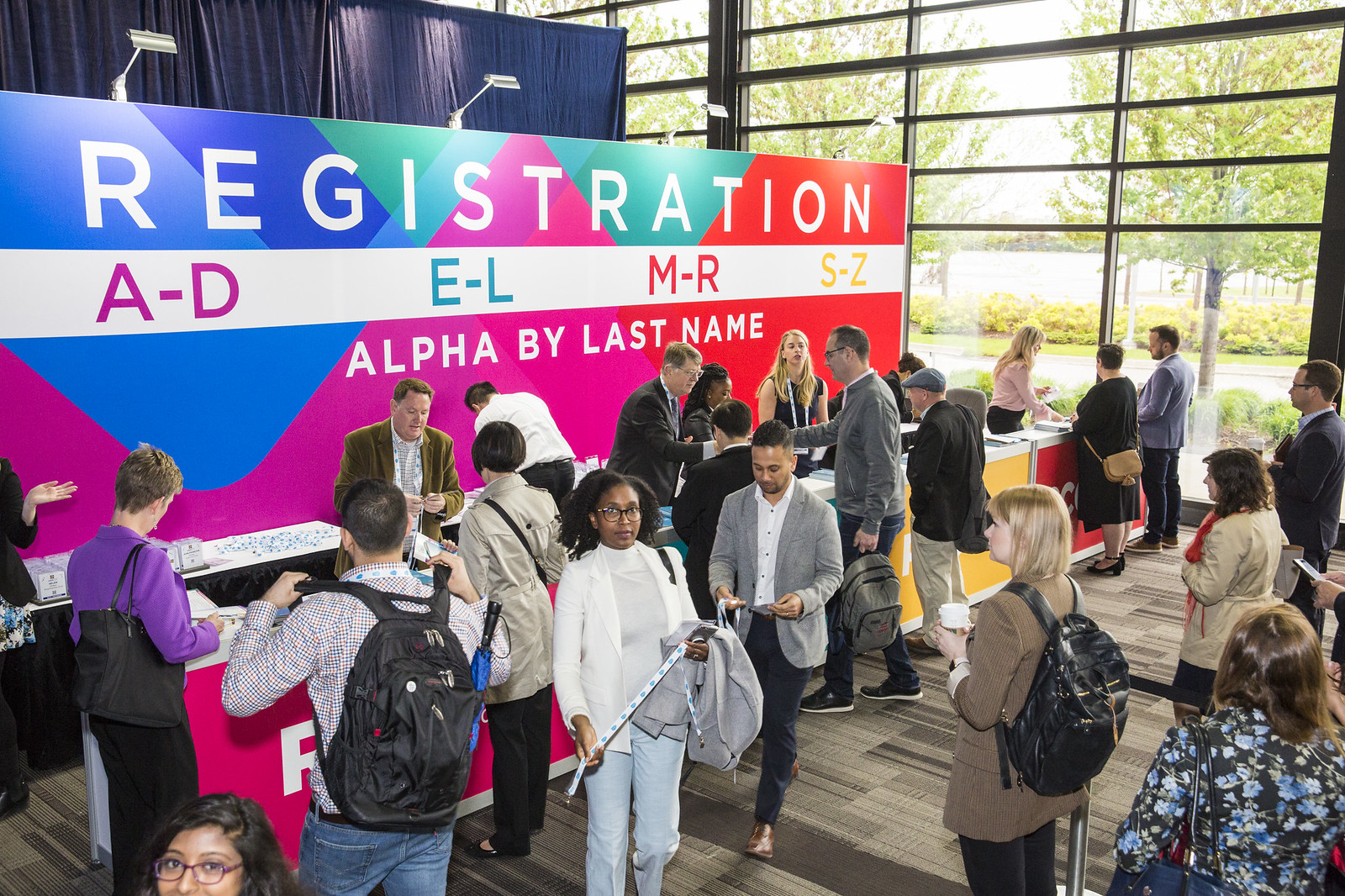This image captures a bustling registration area within a large, well-lit conference room, possibly part of a convention center. The room is filled with adults of various ethnicities and ages, ranging from their late 20s to 50s, who are milling around a long counter-top table divided into several sections for registration, organized alphabetically by last name: A through D, E through L, M through R, and S through Z. Behind the table is a vibrant, multicolored sign with bold lettering that reads "Registration." The background features a wall of large windows with black frames, allowing natural light to pour in and revealing a lush outdoor area with trees. The floor is either wooden or carpeted in gray, adding a touch of elegance to the scene. The ambiance is lively and organized, with people coming and going, some carrying bags and jackets, presumably obtaining their badges for the event. The registration area is brightly lit by four lamps, casting a welcoming glow over the proceedings.